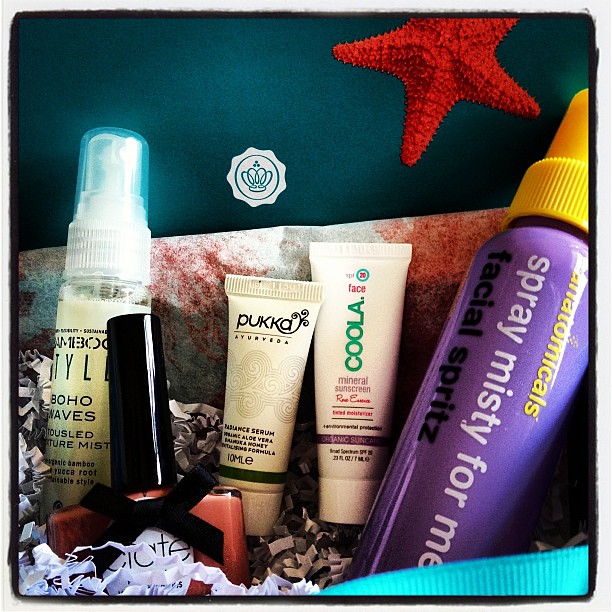This detailed image features an array of personal care products neatly arranged inside a subscription box. The box, which has a dark blue lid with a white sticker adorned with a dark green crown outline and a partially visible red starfish in the top right corner, is filled with crumpled white paper and confetti for padding.

From left to right inside the box, the products are as follows: 
- A white spray bottle with gold-colored liquid.
- In front of this bottle, there's a distinctive nail polish bottle in red or flesh color with a black bow and a tall black shiny cap, featuring a white circle with text 'crate' on the front.
- Centrally located are two white tubes. The first tube reads "Pukka," referring to an Ayurvedic serum with aloe vera, while the second is labeled "COOLA Face," indicating it is a mineral sunscreen.
- On the far right, there's a prominent purple bottle labeled "anatomicals" in yellow, with additional text reading "Spray Misty for Me" in white and "Facial Spritz" in black, topped with a yellow cap.

The entire setup is accentuated with a blue background, giving it a clean and vibrant aesthetic, typical of product photography with a realistic, representational style.